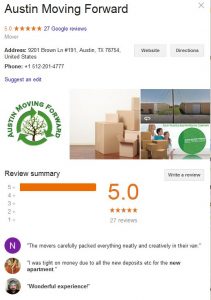Screenshot Caption: Detailed Description of "Austin Moving Forward" Webpage

The image is a screenshot of a webpage or app, specifically showcasing the "Austin Moving Forward" page. The page features a clean, white background, with the main textual and visual elements predominantly aligned to the left.

At the top, the title "Austin Moving Forward" is prominently displayed in large, bold black font. Directly beneath this title, there's a section dedicated to reviews. This section shows a 5-star rating system followed by "27 Google reviews," although the text is slightly blurred and hard to read when zoomed in.

Below the review section, there appears to be an address listed, indicating that the business is located in Austin, Texas, USA, but the specific details are not entirely legible. Accompanying this information is a phone number for contact purposes.

To the right of this address and contact information, there are two gray buttons. While the text on these buttons is blurry, it is presumed that one button links to the website and the other provides directions.

Further down the page, a few photos are displayed. The first photo is likely their logo, "Austin Moving Forward," featuring a green circle with a tree inside against a white background. The second photo depicts moving boxes in an empty room, symbolizing their moving services. The third image seems to be a composite of two photos: one with a family and boxes, possibly indicating a happy customer, and the other with large warehouses, suggesting storage facilities.

At the bottom of the page, there is a review summary section. This summary reiterates the 5-star rating and displays the total number of reviews. Additionally, there is a button to write a review and a few highlighted sample reviews from customers.

Overall, the screenshot provides a comprehensive overview of the "Austin Moving Forward" page, highlighting key information and visual elements that represent the moving and storage services offered by the business.